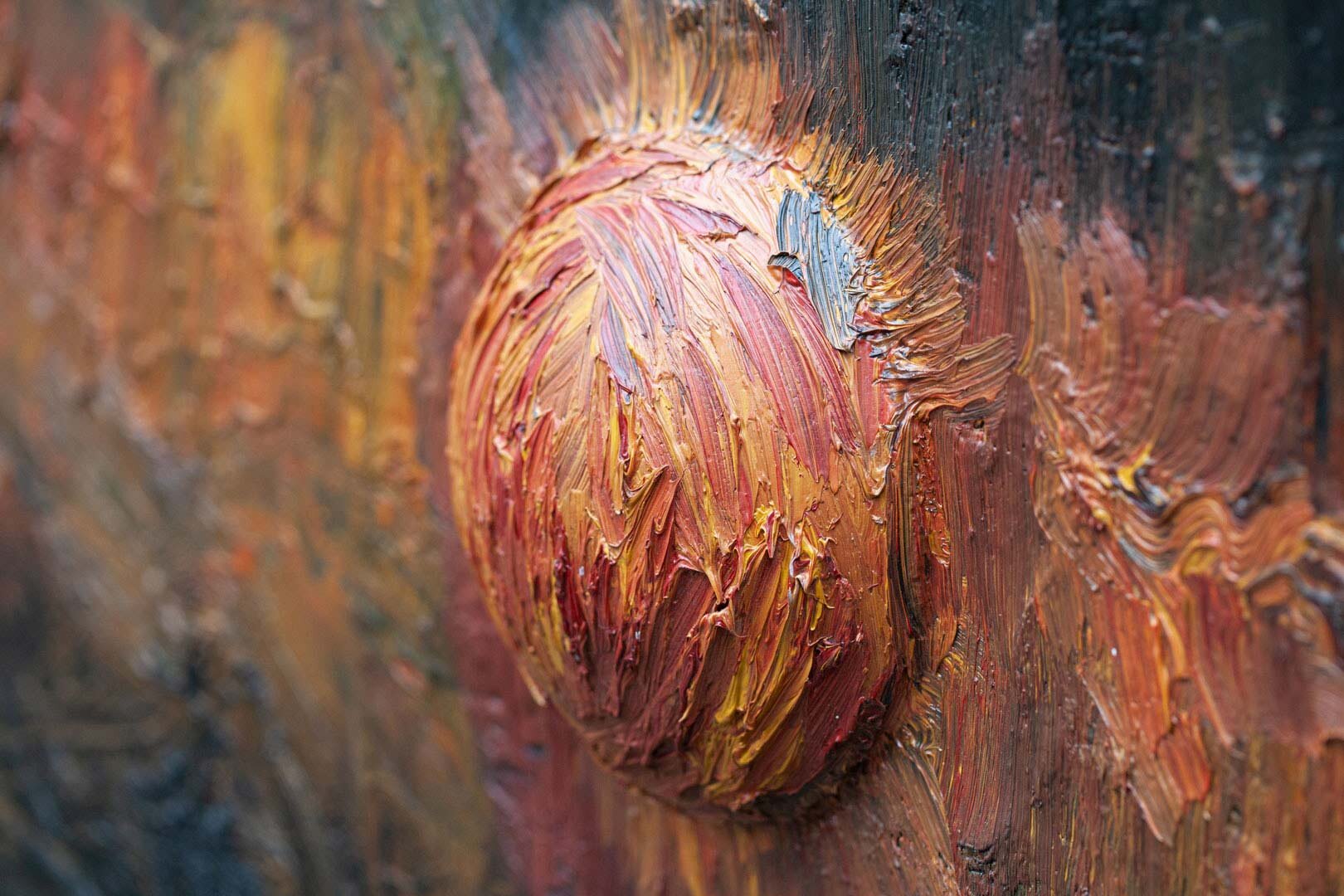The image depicts a highly textured, semi-spherical bulge protruding from a flat, rectangular surface, possibly a canvas, that is thickly layered with vibrant oil paints. The bulge itself, resembling a dome or a wart, is prominently painted in striking hues of pink, blue, yellow, orange, and gray. The artist has applied the paint in such a way that each brush stroke is distinctly visible, creating an intricate pattern of ridges and waves. The overall surface, predominantly painted in red, yellow, orange, and black, extends horizontally across the frame, with portions appearing out of focus towards the left and right edges. A slight sheen atop the bulging area adds a subtle highlight, emphasizing the paint's glossy, tactile quality. The photograph captures the dynamic interplay of colors and textures, presenting a detailed view of this vividly painted bulge against its artistically textured backdrop.